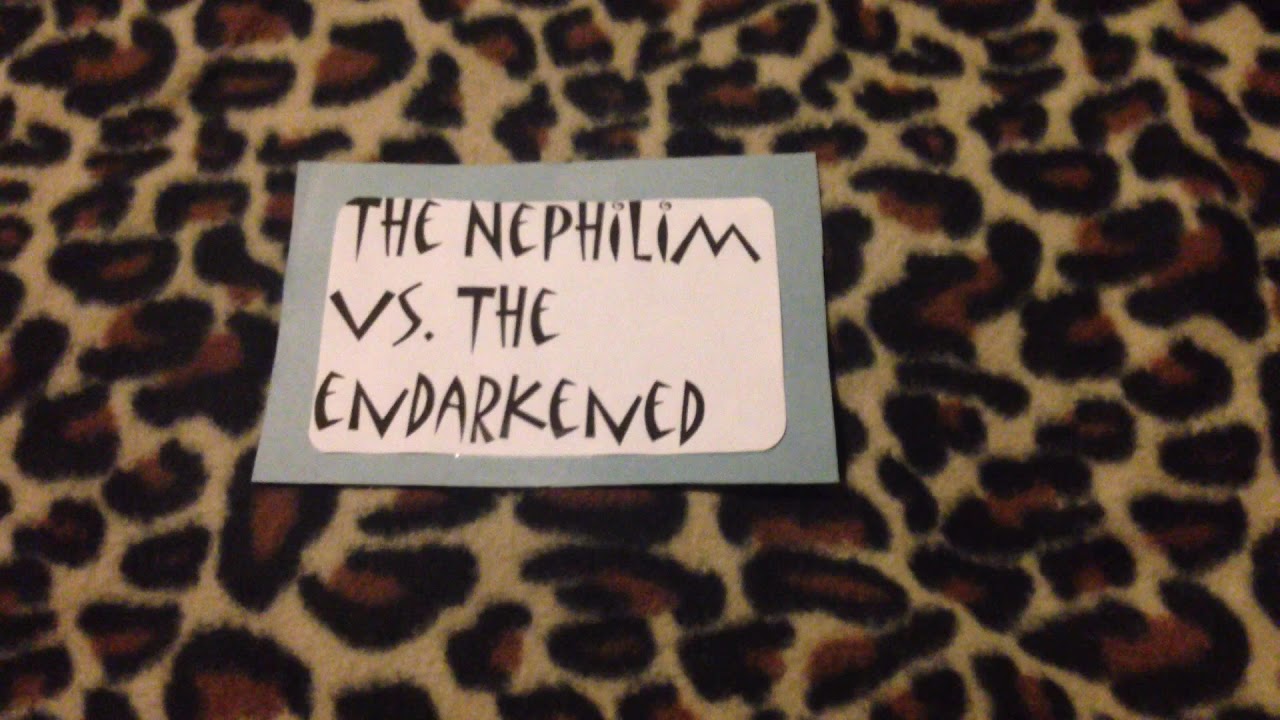In the image, a leopard-patterned background, likely a fuzzy blanket or carpet, displays a striking design with black splotches accentuated by dark brown elements. Set against this vivid backdrop, a gray rectangle, oriented horizontally, centers the composition. Within this gray rectangle is a smaller, white rectangle with rounded edges. In the middle of the white area, elegant and stylized black letters spell out "THE NEPHILIM" on one line and "V.S. THE ENDARKENED" on the next, capturing attention with their bold, all-capitalized font.